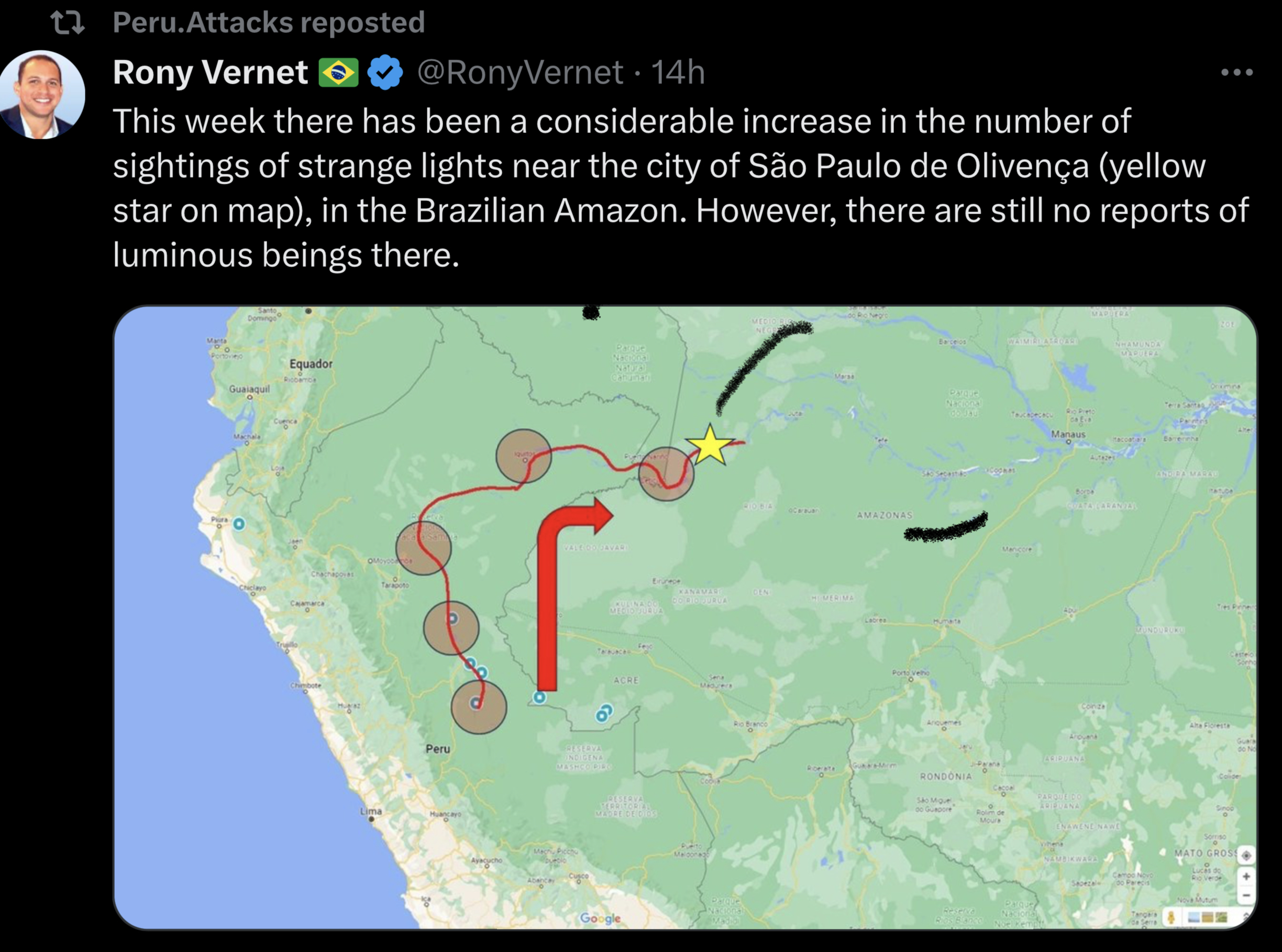Posted by Ronnie Vernet 14 hours ago on X (formerly Twitter), this tweet features a detailed map of Brazil and Peru. The map showcases five circles connected by a squiggly red line, leading to a prominent yellow star at the end. The caption reads:

"This week, there has been a considerable increase in the number of sightings of strange lights near the city of São Paulo, indicated by the yellow star on the map. Despite these numerous sightings, particularly in the Brazilian Amazon region near São Paulo de Olivença, there have been no reports of luminous beings in the area."

Next to Ronnie Vernet's name, you can see a Brazilian flag and a blue checkmark, indicating a verified account. The title above his name says "Peru.Attacks Reposted."